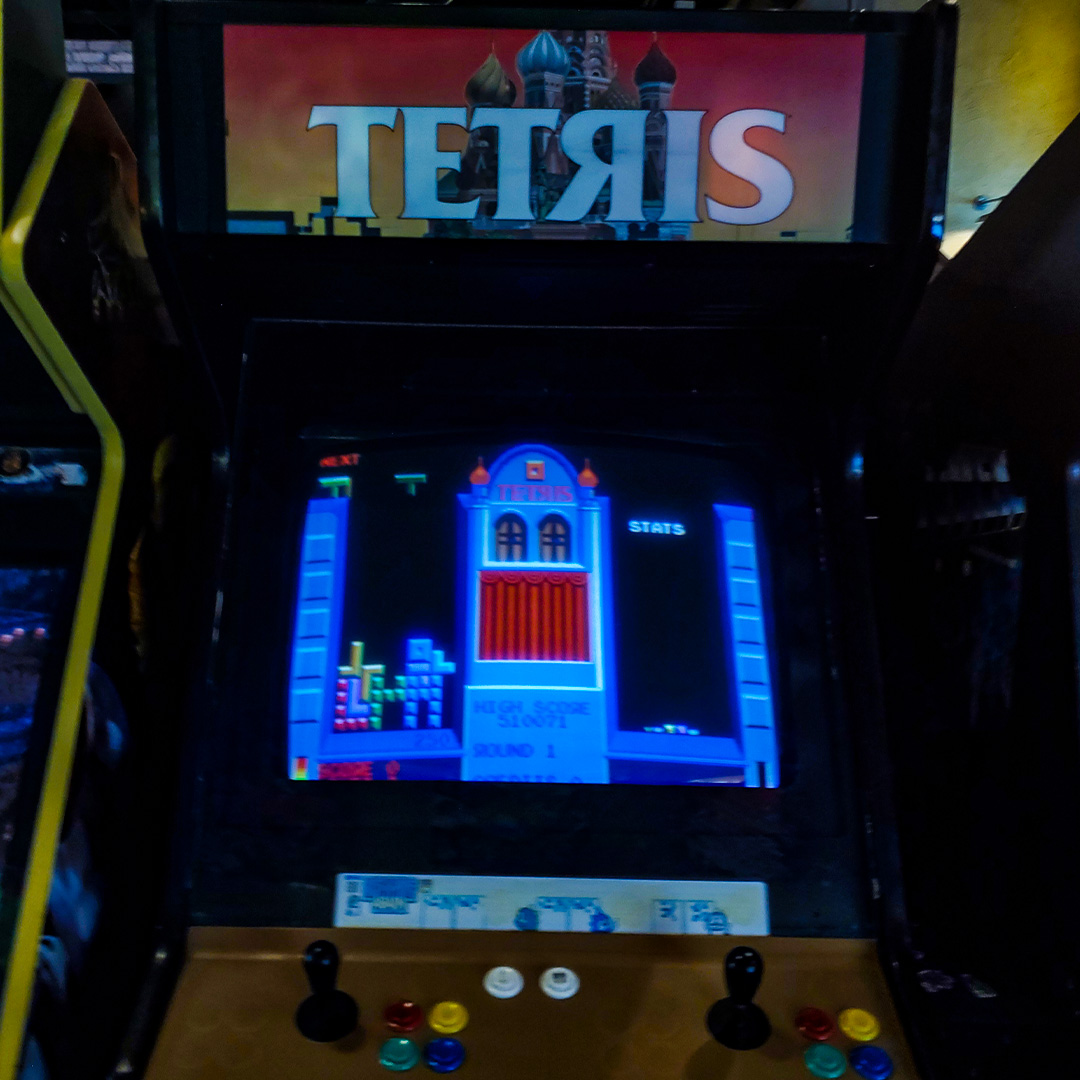This photograph captures an arcade machine with a prominently featured game of Tetris. At the top of the machine, the title "Tetris" is displayed in large white letters, with the R characteristically reversed. Above this, the backdrop showcases the Russian Kremlin building, emphasizing the game's traditional theme. The central screen reveals the gameplay, with colorful Tetris pieces in yellow, orange, black, and green descending against a primarily blue background. The screen displays the game status, with "Stats" in white text on the right.

The control panel below the screen is designed for two players, each equipped with a black joystick. Each player area has a square arrangement of four buttons: a red button at the upper left, a yellow button at the upper right, a blue button at the lower right, and a green button at the lower left. In between the two sets of player controls, there are two white buttons, presumably for selecting the number of players. The first white button is faded, while the second one has a black silhouette image of two people. The setting indicates that only one player seems to be active at the moment, as reflected by the lone set of blocks on the left side of the screen, while the right side shows game statistics.